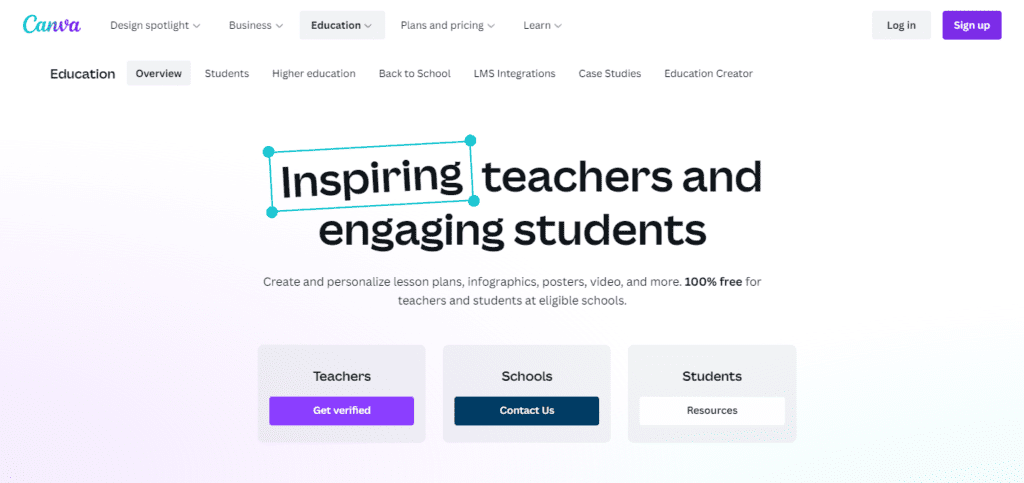The image depicts the homepage of Carwah's website, designed to inspire teachers and engage students. Dominating the center of the page, a bold message in large black letters reads "Inspiring Teachers and Engaging Students." Notably, the word "Inspiring" is slightly slanted and highlighted in a green box with green dots at its corners. The site boasts three main columns for different user categories: teachers, schools, and students. 

Along the top navigation bar, visitors can explore sections including Design, Spotlight, Business, Education, Plans and Pricing, and Learn, each featuring drop-down menus for further options. The Education section's drop-down menu lists links to Education Overview, Students, Higher Education, Back to School, LMS Integration, Case Studies, and Education Creator. 

The website emphasizes its offerings with a statement: "Create and personalize lesson plans, infographics, posters, video, and more. 100% free for teachers and students at eligible schools." 

For teachers, there's an option to get verified, highlighted in a vibrant purple box, while schools have a black box for contacting the company. The section for students, featuring a white box labeled "Resources," ensures that all users have tailored options available. This well-organized platform is evidently a valuable tool for the educational community.